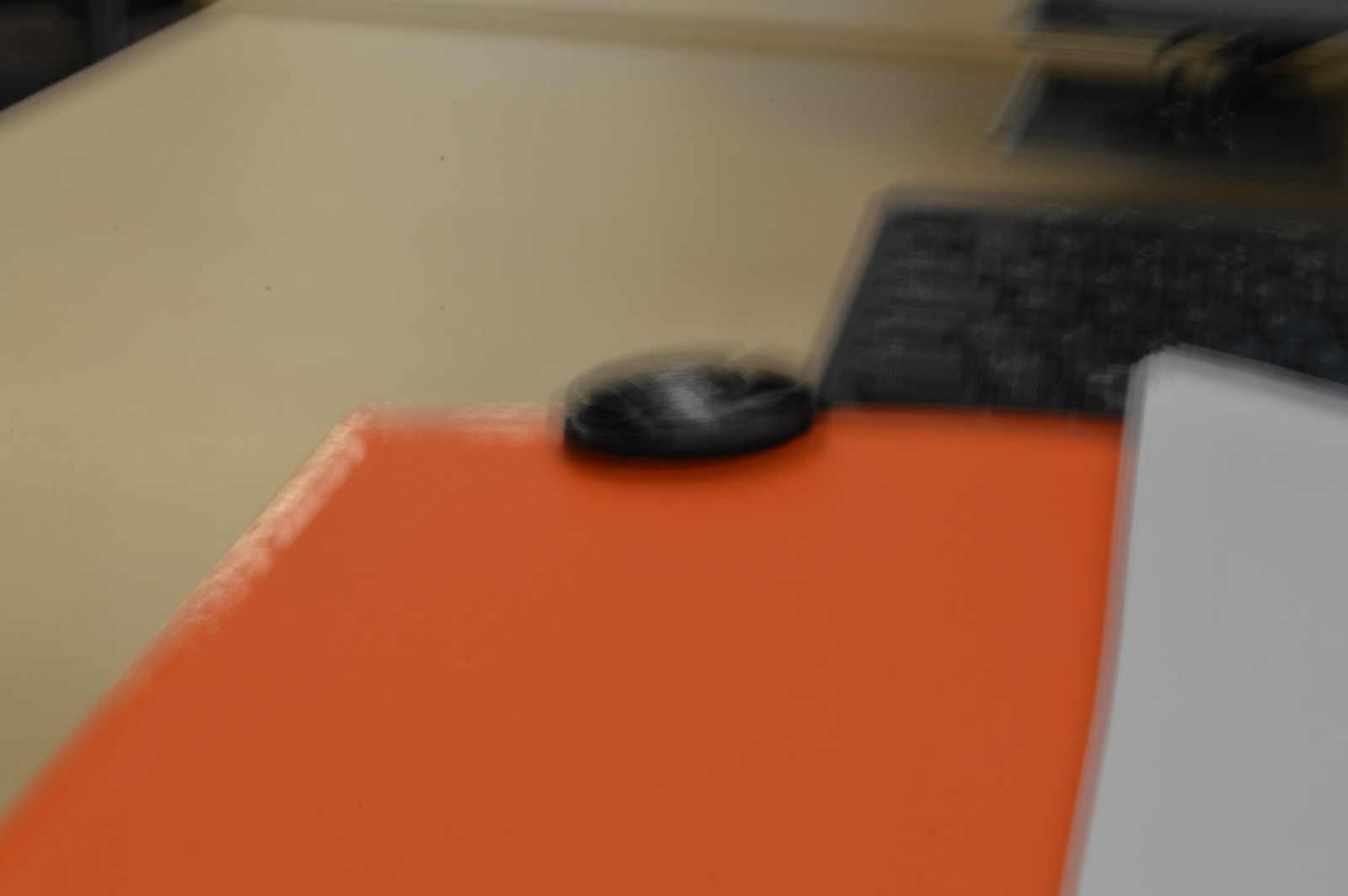This image depicts a blurry scene of a desktop workspace. On the right-hand side, a white object can be observed, which appears to be a binder, resting on an orange surface that exhibits some shiny lining. The desk itself is largely orange in this section, transitioning to a tan color beyond the orange area. In the upper right-hand corner of the image, a keyboard is faintly visible, and right above it, one can discern the base of a monitor. Additionally, there is a black mouse positioned to the bottom left of the keyboard.